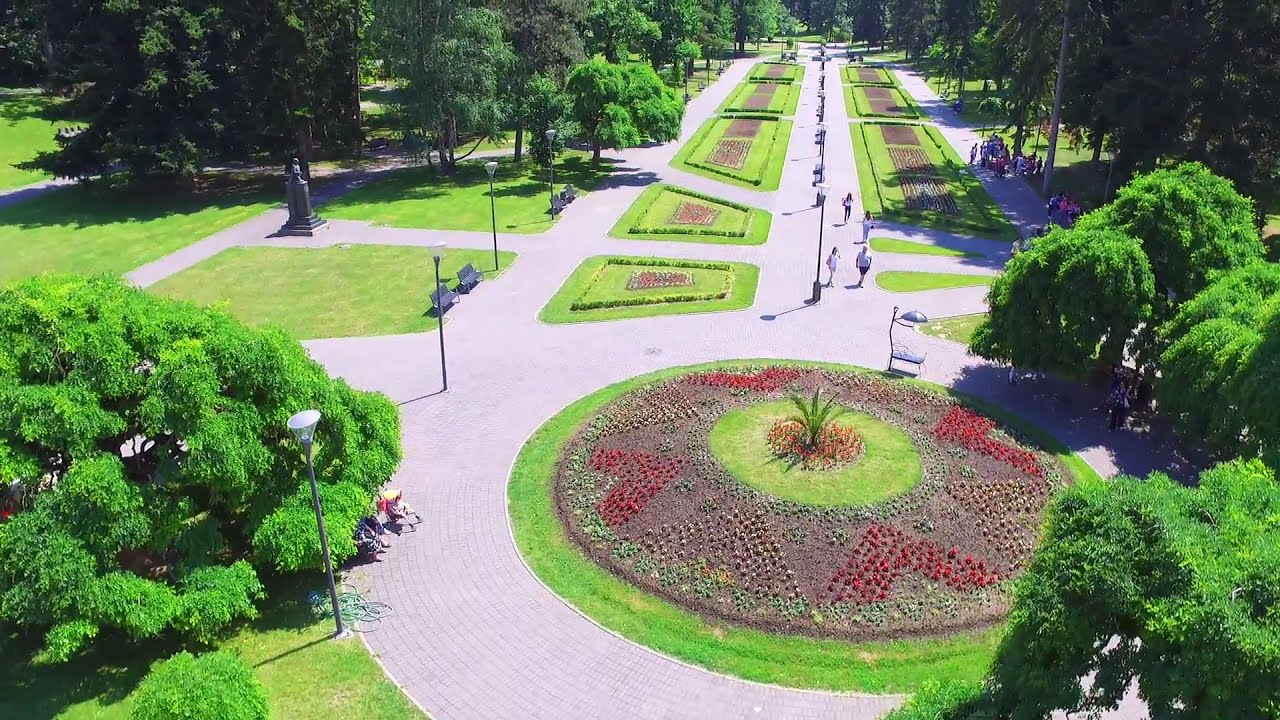This image captures a stunning aerial view of a beautifully landscaped public park, showcasing an intricately designed central garden. At the heart of the park is a circular garden adorned with vibrant red plants arranged in shapes that appear like hearts on all sides. A light green fern-like plant flourishes at the center. This circular garden is encircled by a brick or stone pathway, adding an elegant touch.

Surrounding the main circle are various rectangular and square garden plots, each neatly organized with diverse plants and flowers that contribute to a mosaic of colors and patterns. Beyond the central garden, a primary pathway extends upward, flanked by smaller brick or white stone paths to the right and left. The pathways, equipped with regularly spaced lampposts, provide ample seating with benches, and the sunny daytime setting shows people walking and relaxing throughout the area.

On the left side of the image, a large tree provides shade for two babies in strollers. The park's lush, green grass and numerous trees in the background enhance the serene and picturesque ambiance, making it an inviting retreat for visitors.